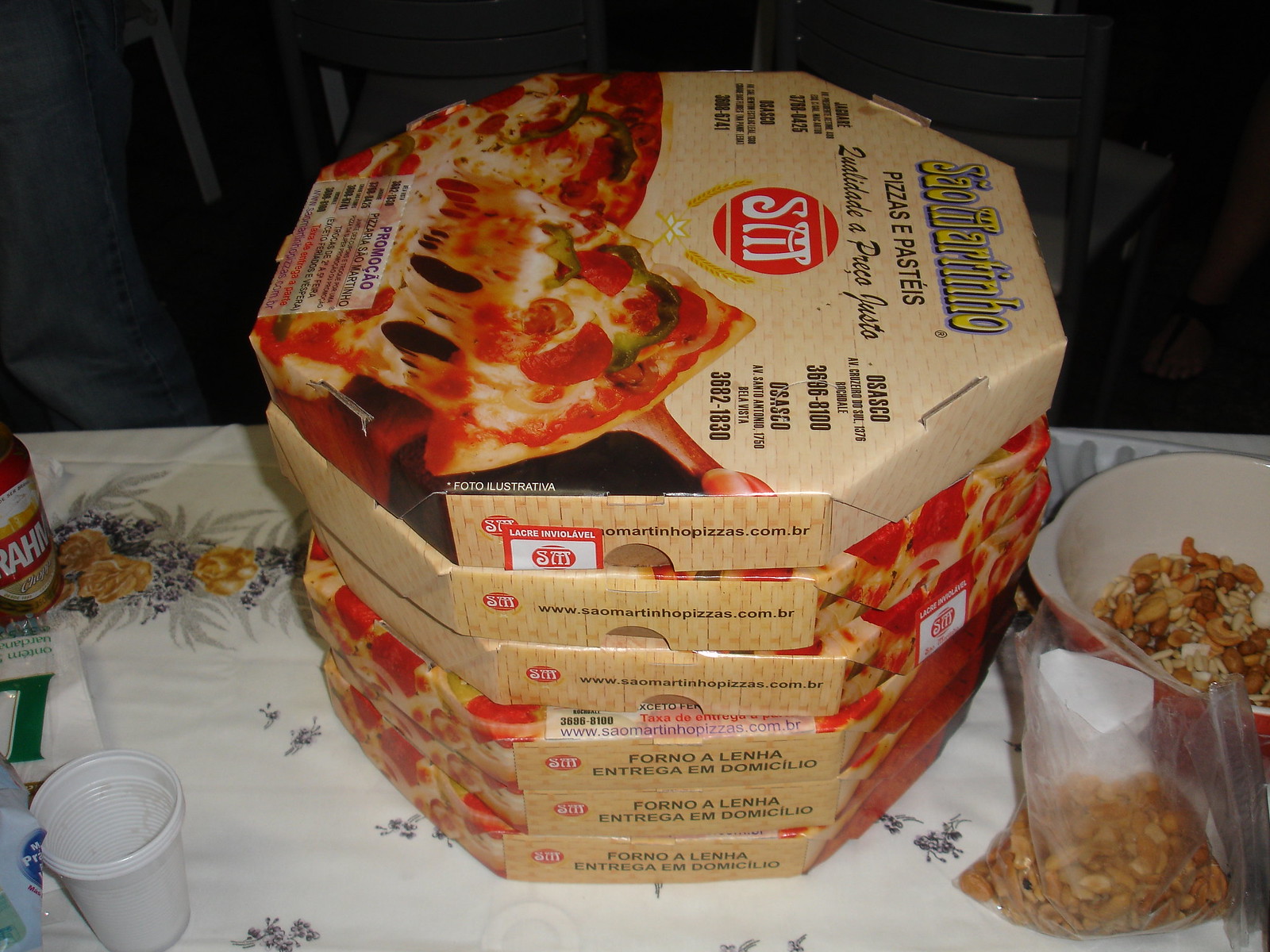The photograph features a stack of six large octagonal pizza boxes, prominently displayed at the center. These boxes, brown in color, showcase an image of a pepperoni pizza with green peppers, highlighting a slice being taken out on the front cover. The packaging features a red logo with white "SM" lettering in the middle, and the brand name "Sal Martino" scripted in yellow at the top. Below the name, the phrase "Pizzas e Pastas" is printed in black, indicating an Italian brand. The sides of the pizza boxes display the URL "www.saomartinopizzas.com.br." The boxes rest on a white tablecloth adorned with blue and gold floral patterns. To the right of the stack, there is a bag and a bowl filled with a snack mix. Additionally, on the top left of the photo, there are a plastic cup, some plastic utensils, and a partially visible bottle.